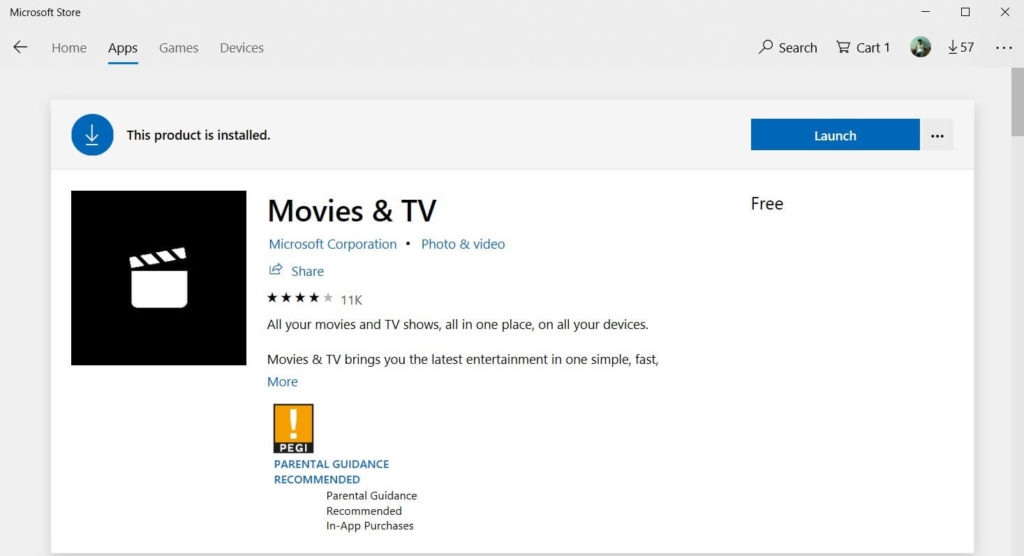This detailed caption was cleaned up and formulated:

---

A screenshot from the Microsoft Store interface displays a horizontal rectangular image with a light gray background. Within this area, there is a smaller white box featuring a light gray ribbon across its top.

Starting with the main light gray background, the upper left corner showcases "Microsoft Store" written in black text. Below this, navigation options are listed: a back arrow, Home, Apps (highlighted in black indicating it is selected), Games, and Devices (all in light gray text).

On the right-hand side, icons for search (magnifying glass), a shopping cart with one item in it, the user's profile picture within a circle, and a download icon displaying the number 57 to its right are visible. The top corner also includes window control buttons: minimize, maximize, and close.

Inside the smaller white box, a gray banner at the top contains a download icon within a navy blue circle, where the icon itself is white. To the right of this, bold black text reads "This product is installed." At the far right of this section, there is a navy blue button with "Launch" written inside in white text, followed by three horizontal dots indicating more options.

Within the white box content, a small black square contains a director's board icon in white. Next to this, bold black text states "Movies & TV." Below this, smaller bright blue text reads "Microsoft Corporation Photo & Video" followed by a "Share" link also in bright blue. A star rating indicating four stars with 11,000 reviews is displayed beneath this text. An additional black text caption reads "All your movies and TV shows, all in one place on all your devices. Movies & TV brings you the latest entertainment in one simple fast…" which is cut off, with "More" written in bright blue suggesting additional content is available.

---

This updated caption provides a structured and detailed description of the screenshot's content from the Microsoft Store interface.